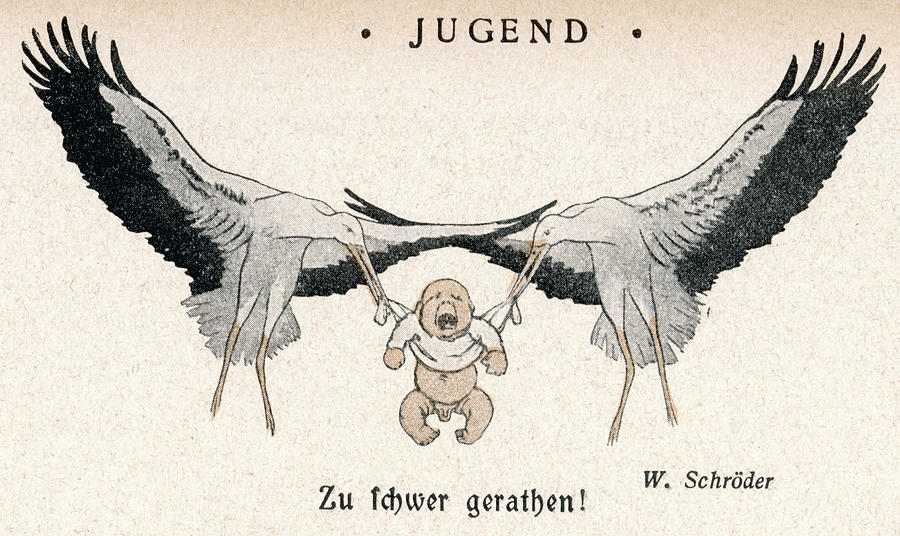This image, rendered in an old, weathered drawing style, features a detailed and expressive scene set against a light pink backdrop dotted with grayish-blue spots. At the top, in black capital letters flanked by black dots, the word "JUGEND" is prominently displayed. Below this, two storks in mid-flight dominate the scene, their outstretched wings overlapping slightly. Their white bodies contrast with the black tips and bottoms of their wings, as well as their yellow beaks and legs which hang below. Each stork delicately holds a corner of a white long-sleeved shirt with their beaks, supporting a crying, nearly naked baby with distinctly visible fingers, toes, and a clear indication that the baby is a boy. The baby dangles precariously as he is carried through the air. At the bottom right, the name "W. Schroeder" is inscribed, and beneath the baby, some German words are visible, likely saying something akin to "Zootochila geronten." The entire composition evokes a sense of vintage artistry encapsulated in a scene of surreal charm and slight distress.